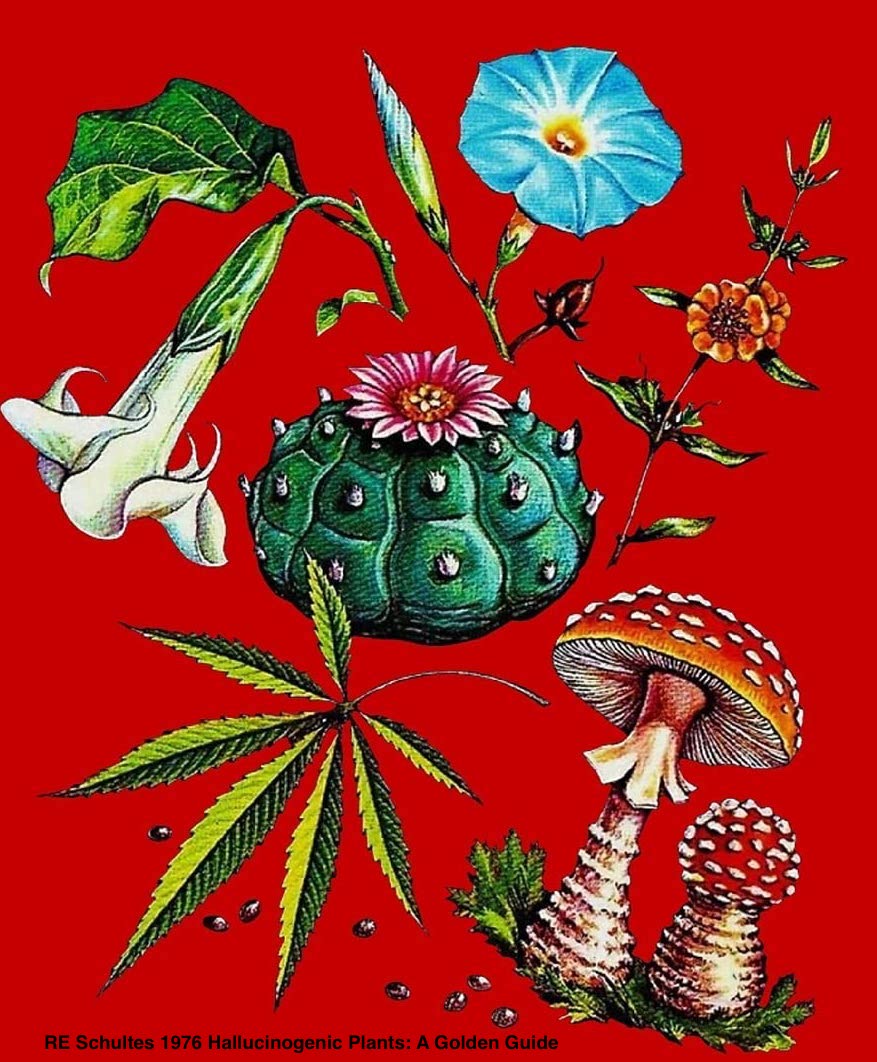The book cover is richly illustrated and appears to be done in acrylic paint. The predominant background color is red. At the bottom, the text reads "R.E. Schultes, 1976, Hallucinogenic Plants, A Golden Guide." The illustration showcases various hallucinogenic plants, vividly depicted. In the center, there is a squat green cactus with a striking pink flower on top. To the bottom right of the cactus, two red toadstools with white spots are shown. In the top left corner, there's a tubular white flower accompanied by a large green leaf. Adjacent to this, a blue morning glory flourishes, complemented by a smaller unopened bud. Nearby is a stem bearing two orange flowers. On the right side of the cover, a distinctive green marijuana leaf is prominently featured. The artwork is vibrant and meticulously detailed, emphasizing the wide range of colors and textures of these hallucinogenic plants.